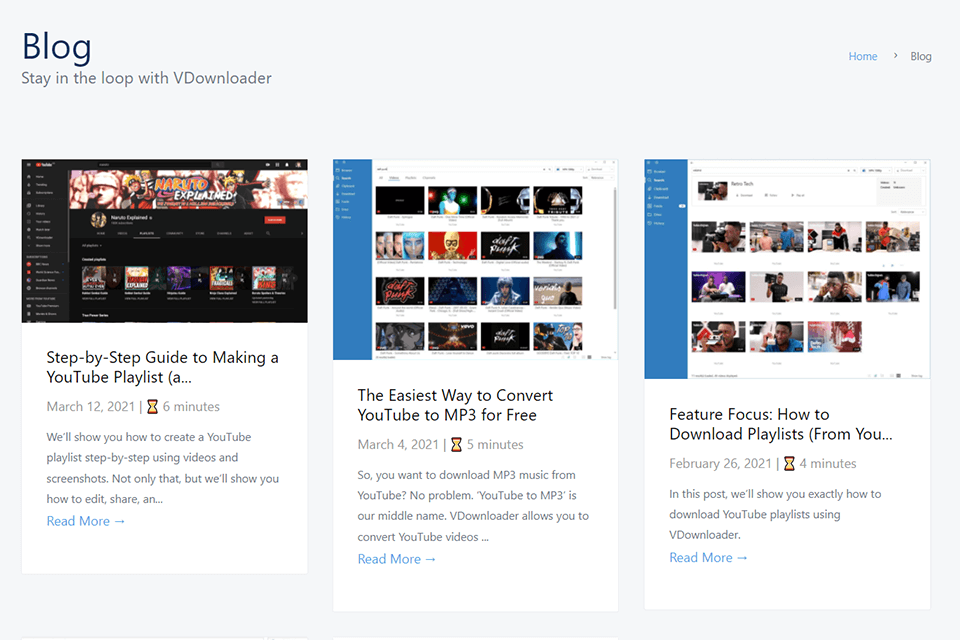This is a detailed screenshot of a webpage, prominently displaying a blog section dedicated to VDownloader. 

At the top left corner, a label reads "Blog - Stay in the loop with VDownloader," indicating the page’s focus on keeping users informed about the tool’s features. On the top right, a navigation breadcrumb shows "Home > Blog," providing users a clear pathway back to the homepage.

Below this header, there are three featured blog posts, each accompanied by a corresponding image and a brief description. 

1. The first image is a screenshot of a YouTube page with a video titled "Naruto Explained." The blog post beneath this image is titled "Step-by-Step Guide to Making a YouTube Playlist" and is dated March 12, 2021. The post promises a 6-minute tutorial on creating a YouTube playlist, including editing and sharing tips. Although the description gets cut off, a "Read more" link is available for further reading.

2. The second image displays multiple YouTube video thumbnails. The associated blog post is titled "The Easiest Way to Convert YouTube to MP3 for Free," dated March 4, 2021, with a 5-minute read time. The description hints at a guide on downloading MP3 music from YouTube, emphasizing VDownloader’s capability for converting videos. A "Read more" link invites users to delve deeper into the article.

3. The final image also showcases an array of YouTube video thumbnails. This post, titled "Feature Focus: How to Download Playlists from YouTube," is dated February 26, 2021, and promises a 4-minute read. The truncated description suggests detailed instructions on using VDownloader to download YouTube playlists. A "Read more" link offers further information.

Each post is geared towards educating users on maximizing VDownloader’s features, ensuring a comprehensive and user-friendly experience.